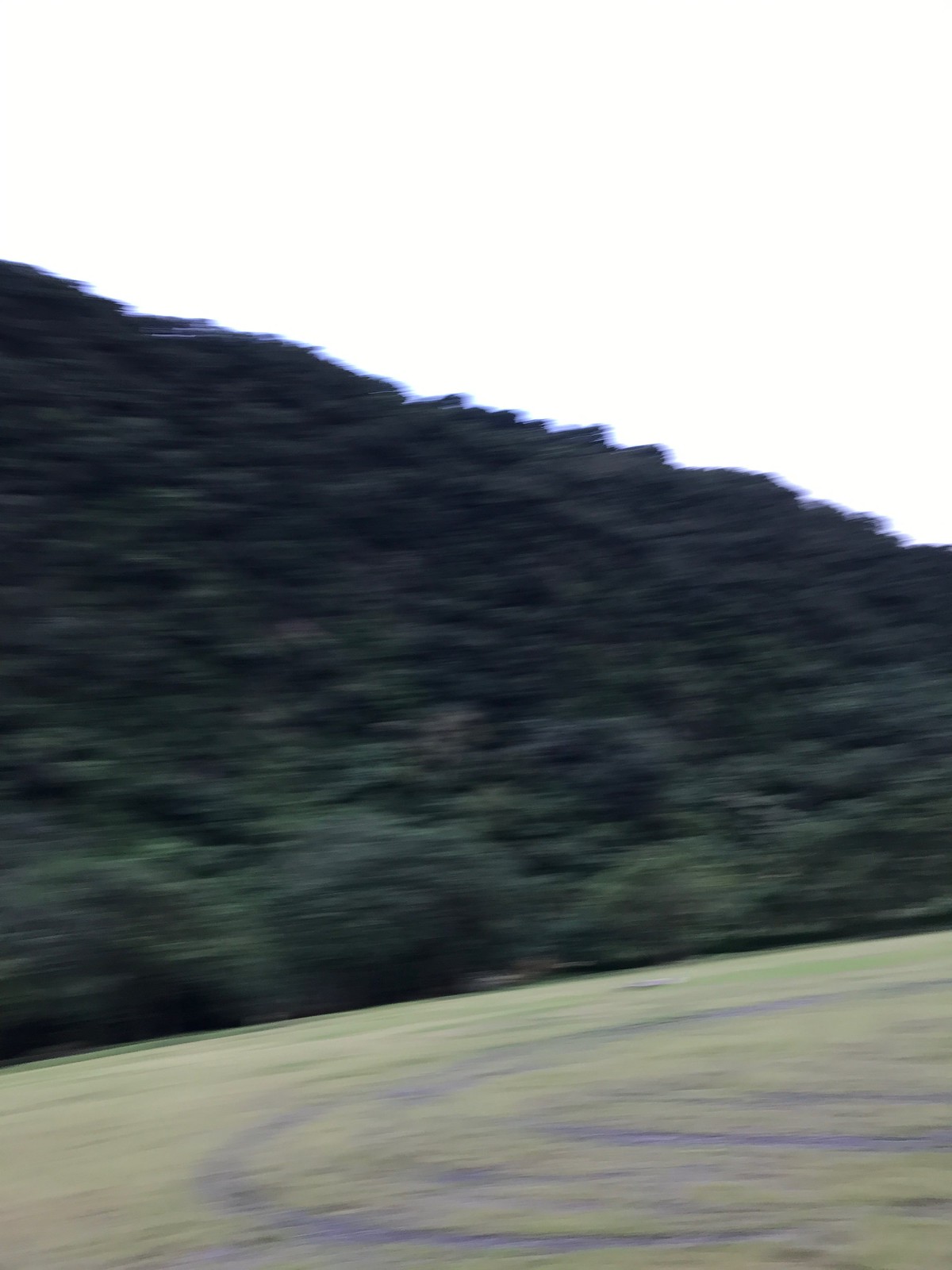This is a blurry daytime photograph of a serene landscape under an overcast sky, which appears white and slightly darkened. The horizon is defined by a hill that rises on the left and gently slopes down towards the right. The hillside is densely populated with mostly deciduous trees, forming a lush green canopy, and is bordered at its base by smaller green bushes. In the foreground lies a flat, predominantly tan area interspersed with patches of green, suggesting a mixture of grass and earth. There is a small, curving section of a track, colored in a bluish-purple hue, partially visible. This narrow loop might belong to a jogging or horse track, although its exact purpose is uncertain. Additional lines of the same color and more grass are discernible within the track area, adding texture to the scene.